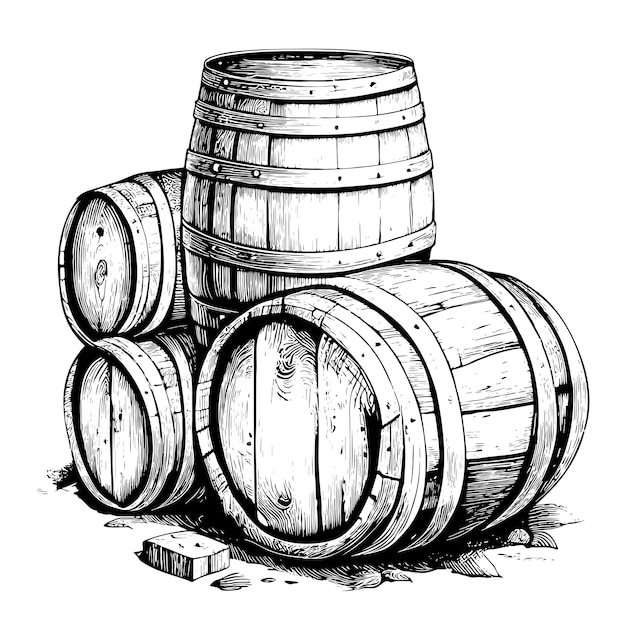This black and white ink sketch showcases four wooden barrels against a solid white background. The barrels are substantial in size, with one standing upright and three lying on their sides. The largest barrel, closest to the viewer, lies on its side, slightly tilted to the left, featuring two horizontal bands and a band on both the top and bottom. Positioned to the left and extending away from the viewer, two more barrels rest on their sides, also slightly angled to the left. Between these barrels and the largest one, an upright barrel is situated, adorned with three horizontal bands. Below the barrels, there appears to be a depiction of grass, and in front of the largest barrel, there's a small chunk of wood. The entire composition is set upon a detailed, monochrome background, and stones can be seen beneath the barrels, adding texture to the scene. The white background dominates the visual space, emphasizing the intricate black and white artwork.